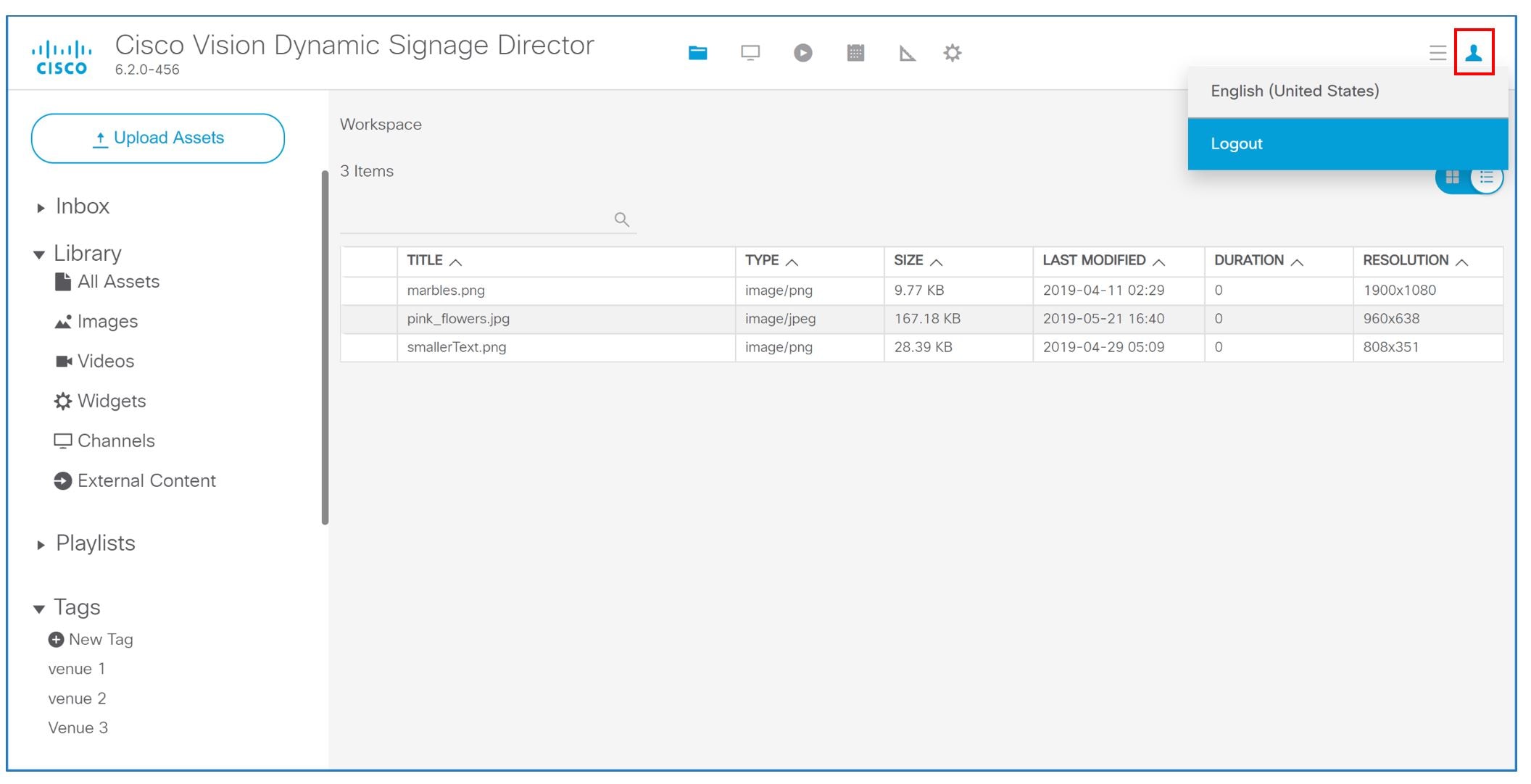This screenshot captures the interface of the "Cisco Vision Dynamic Signage Director" app, taken from a computer screen. The user is preparing to log out, as indicated by a red box highlighted over the user icon and the "Log Out" option selected beneath "English (United States)" in the language settings. The interface displays the capability for users to upload images, evidenced by the presence of three uploaded images named "marbles," "pink flowers," and "smaller text." Each image is a PNG file approximately 9.77 kilobytes in size, last modified in 2019. Although the actual images are not visible, their file details are provided. The resolution of these images is indicated to vary slightly, with "marbles" having the highest resolution. On the left side of the interface, there is an option for uploading additional assets or images, showing the app's functional layout. The overall design and controls suggest a robust platform for managing and uploading digital signage content.